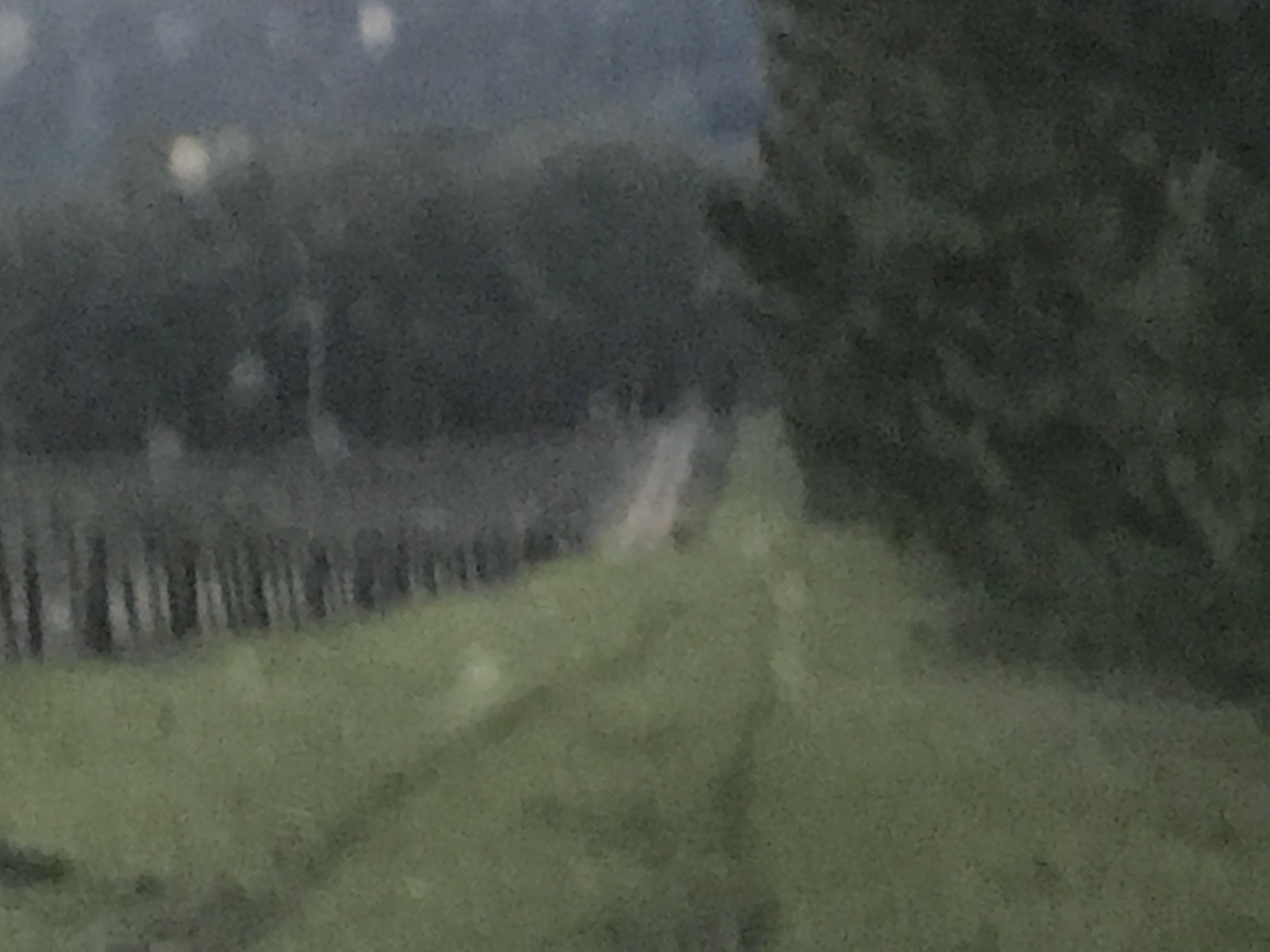A blurry photograph capturing an outdoor scene with a dark, subdued ambiance. A narrow pathway, possibly fit for a tractor or four-wheelers, meanders alongside an old, wooden fence. Large, bush-like trees densely populate the area, partially concealing the pathway. The background is filled with more trees, suggesting a rural setting, possibly near a farm. The overall image is enveloped in a shadowy, dim light, giving it a somewhat gloomy and indistinct appearance. The ground is covered in grass, with no clear indicators of a gravel or dirt road.